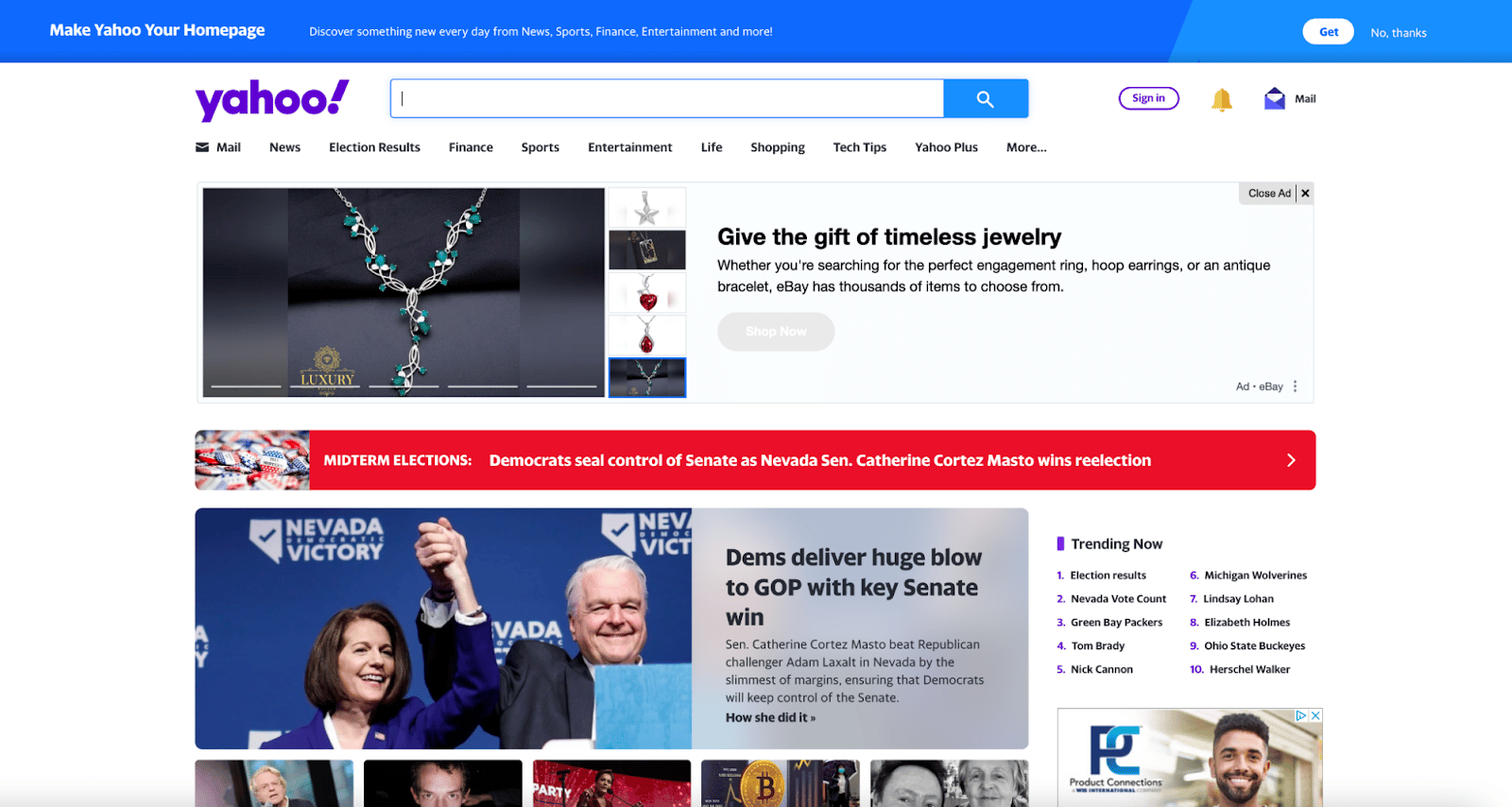This is a cropped screenshot of the Yahoo homepage. At the top, a blue header prompts users to "Make Yahoo your homepage." To the right of this message, there are small white letters, with a tiny white button that says "Get" in blue letters, and next to it, the words "No thanks" in very small white letters.

Below this header is the main Yahoo homepage against a white background. On the left, the "Yahoo" logo is displayed in purple, accompanied by a large, centrally-aligned search bar. To the right of the search bar, there is a small button for "Sign In," outlined and written in purple. Further to the right, a gold bell icon indicates alerts, next to which is a blue envelope icon labeled "Mail."

Beneath the search bar, categories are listed horizontally. Below these categories, a substantial advertisement promoting jewelry gifts features a thumbnail image of jewelry. The ad is marked with a small gray box in the top right corner that says "Ad."

Underneath the ad, a red banner headline announces, "Midterm elections: Democrats seal control of senate as Nevada Senator wins re-election." Another article follows, titled "Tim's delivered huge blow to GOP with key Senate win," displaying a thumbnail image to the left and the article title within a gray box to the right of the photo.

At the bottom-right corner of the screenshot, there is a small box labeled "Trending Now," listing 10 trending topics in tiny black writing. The top part of another ad is visible at the very bottom of the image, but the rest has been cropped out.